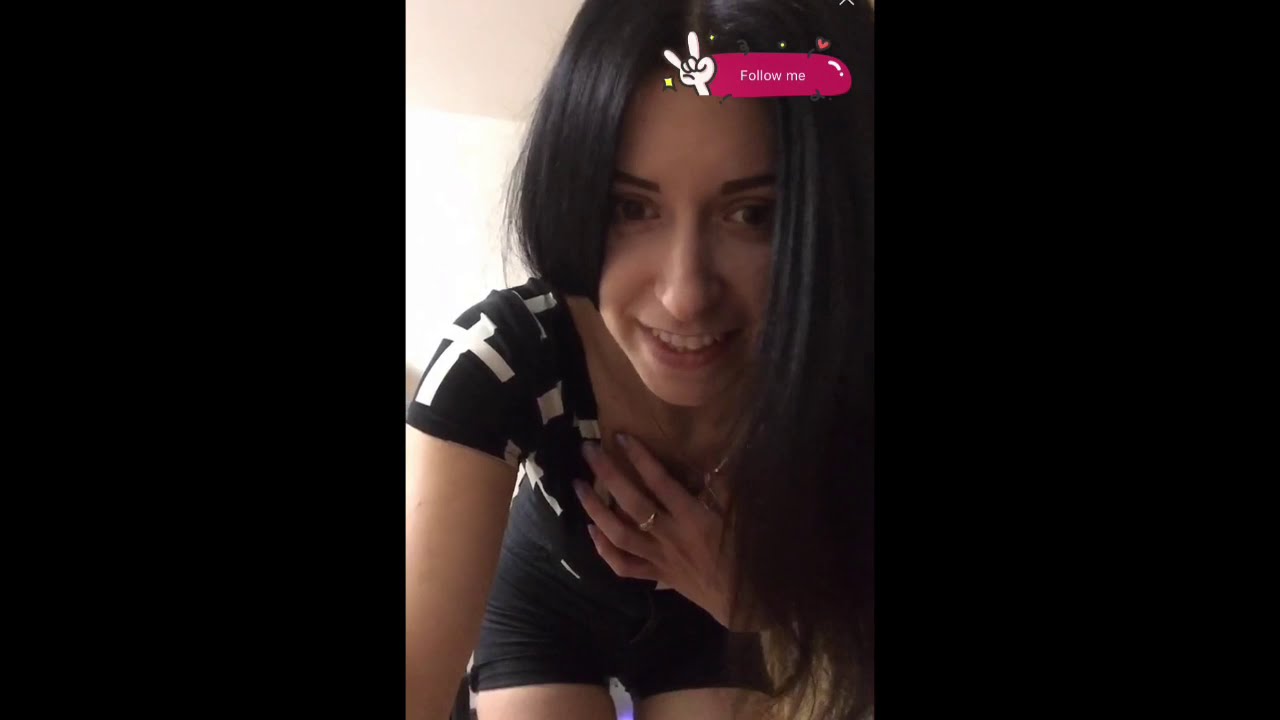This is a detailed photograph featuring a young woman captured in an indoor setting, oriented in portrait mode. The image is structured in three vertical panels, with the middle panel prominently displaying the woman while the left and right bars are plain black.

In the central panel, the woman is leaning slightly forward with her hand across her chest, partially covering herself. She is wearing a black top with white crosses and tight black shorts, visible up to her knees. Her dark, long hair falls partly over her face and hand on the right side, while it is tucked behind her back on the left. She has fair skin and is smiling, revealing her white teeth, with a long, thin nose highlighted in the shot. Notable accessories include a ring on her middle finger and a partially visible necklace around her neck.

The background behind her is white, and in the top right corner, there's a distinct pink oval-shaped box with the words "Follow Me" in white text. Accompanying this text are cartoonish icons: a peace sign hand and small hearts.